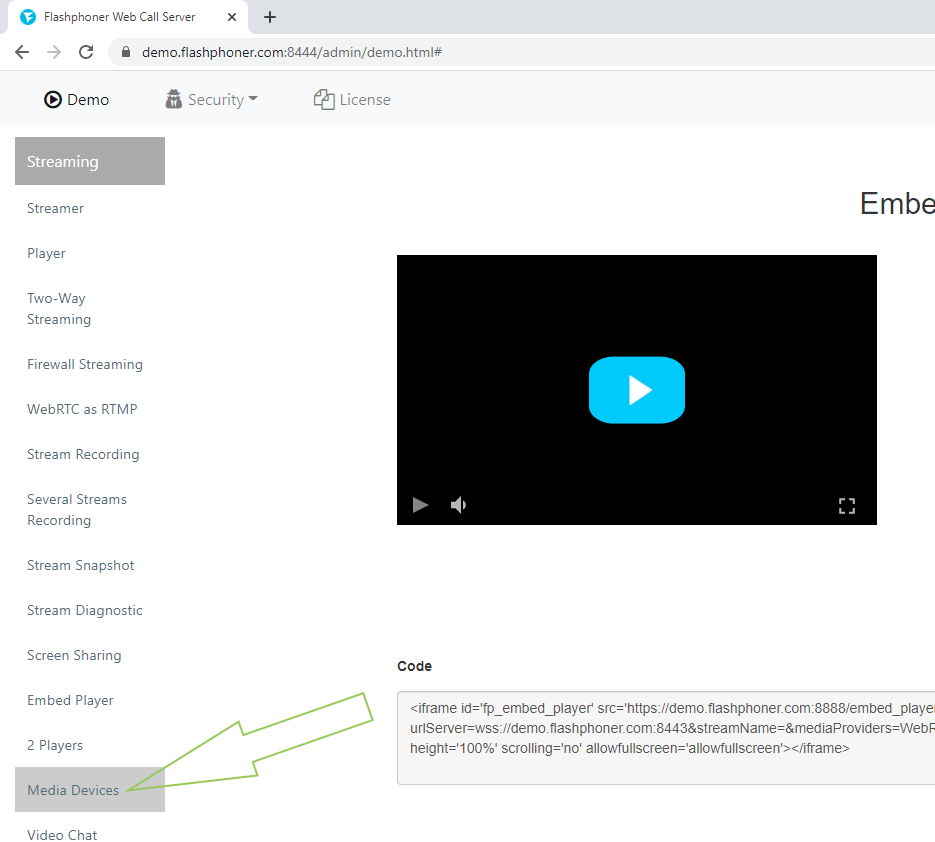The image depicts the user interface of the Flash Phoner Web Call Server. At the top-left corner, within a horizontal rectangle, is the header labeled "Flash Phoner Web Call Server." Below this, there's a text field designated for an URL, displaying "demo.flashphoner.com:8444/admin/demo.html#".

Underneath the URL field, another line is labeled "Demo Security and License." On the left side of the image, there's a vertical column with various options listed: Streaming, Steamer, Streamer, Player, Two-Way Streaming, Firewall Streaming, WebRTC as RTMP, Stream Recording, Several Streams Recording, Stream Snapshot, Stream Diagnostic, Screen Sharing, Embed Player, Two Players, Media Devices, and Video Chat.

An outlined green arrow points downwards towards "Media Devices," originating from the URL field. The URL field itself is within a rectangular box. To the right of this layout is a small, black, square-shaped computer screen. In the center of this screen, there is a turquoise box with a forward arrow drawn in white, signifying an action button or a play icon.